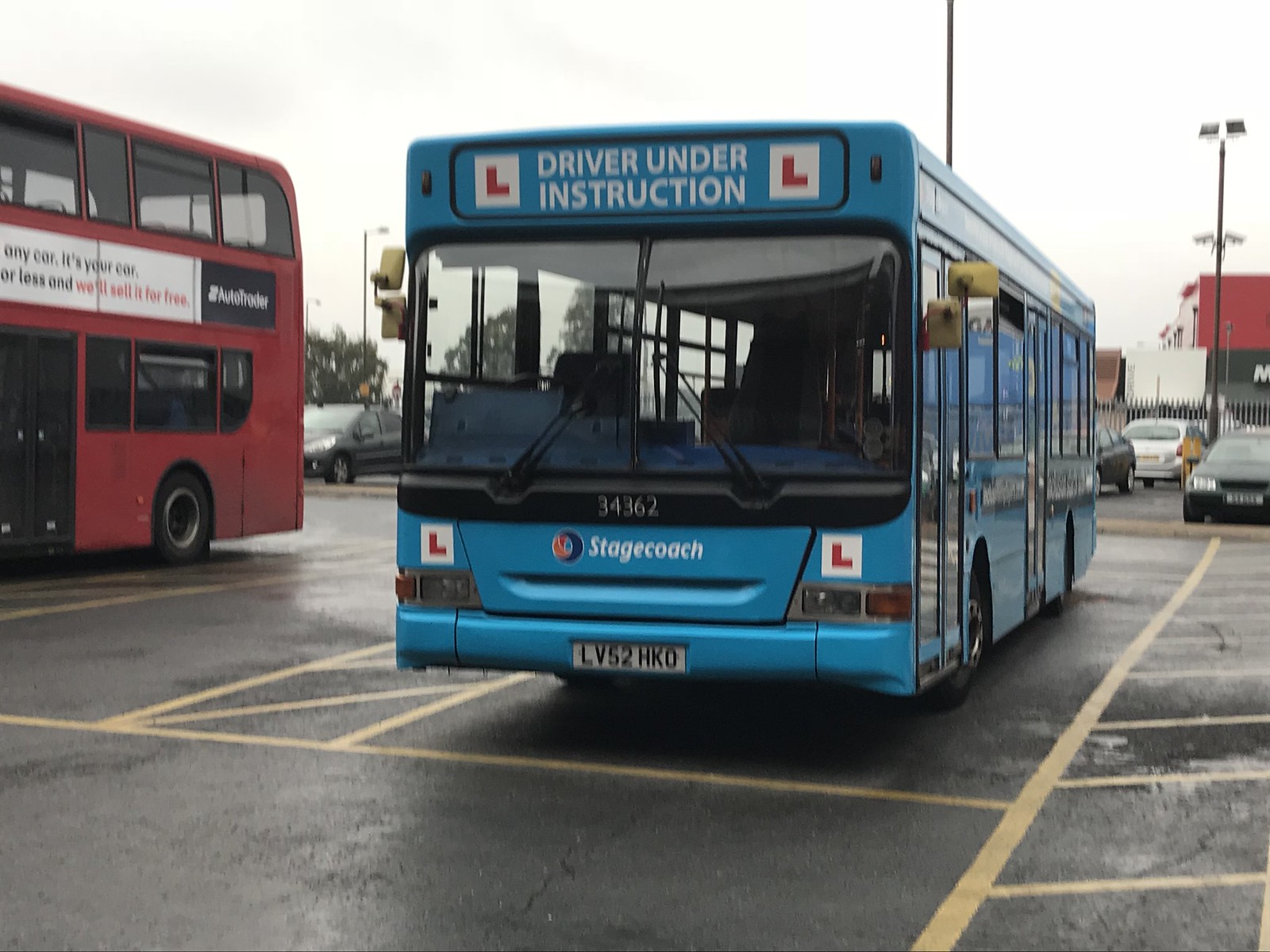The photograph captures a slightly blurry, overcast daytime scene of a blue Stagecoach bus parked in a yellow-lined space on a black, possibly wet, concrete lot. The bus prominently displays the text "DRIVER UNDER INSTRUCTION" in white letters at the top of the front window, flanked by red L plates in white squares. The Stagecoach branding, along with the number "34362," is visible under the driver's window, along with a white European license plate at the bottom edge. To the left of the blue bus, a red double-decker bus with white signage is partially visible. The background includes other parked vehicles and streetlights, against a completely white sky, amplifying the sense of an overcast day.